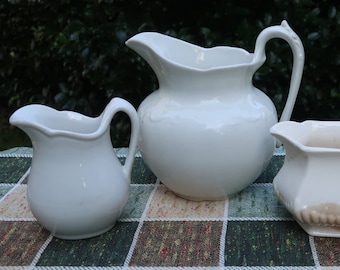The image showcases three ceramic jugs arranged on a flat, tiled surface that features a brown and gray square-shaped pattern. All three jugs share a white base color, but the jug on the right has a slightly cream or beige hue and a brown base. This jug also stands out due to its geometric edges. The central jug, which is the largest, features a spout and a ball-like or curved surface with a wide mouth, making it appear almost circular. To the left of this central jug is a smaller one that mirrors its shape but in a more compact form. They are all glossy, adding a polished touch to their ceramic style. The background of the image is dark, which accentuates the jugs’ bright, shiny surfaces.